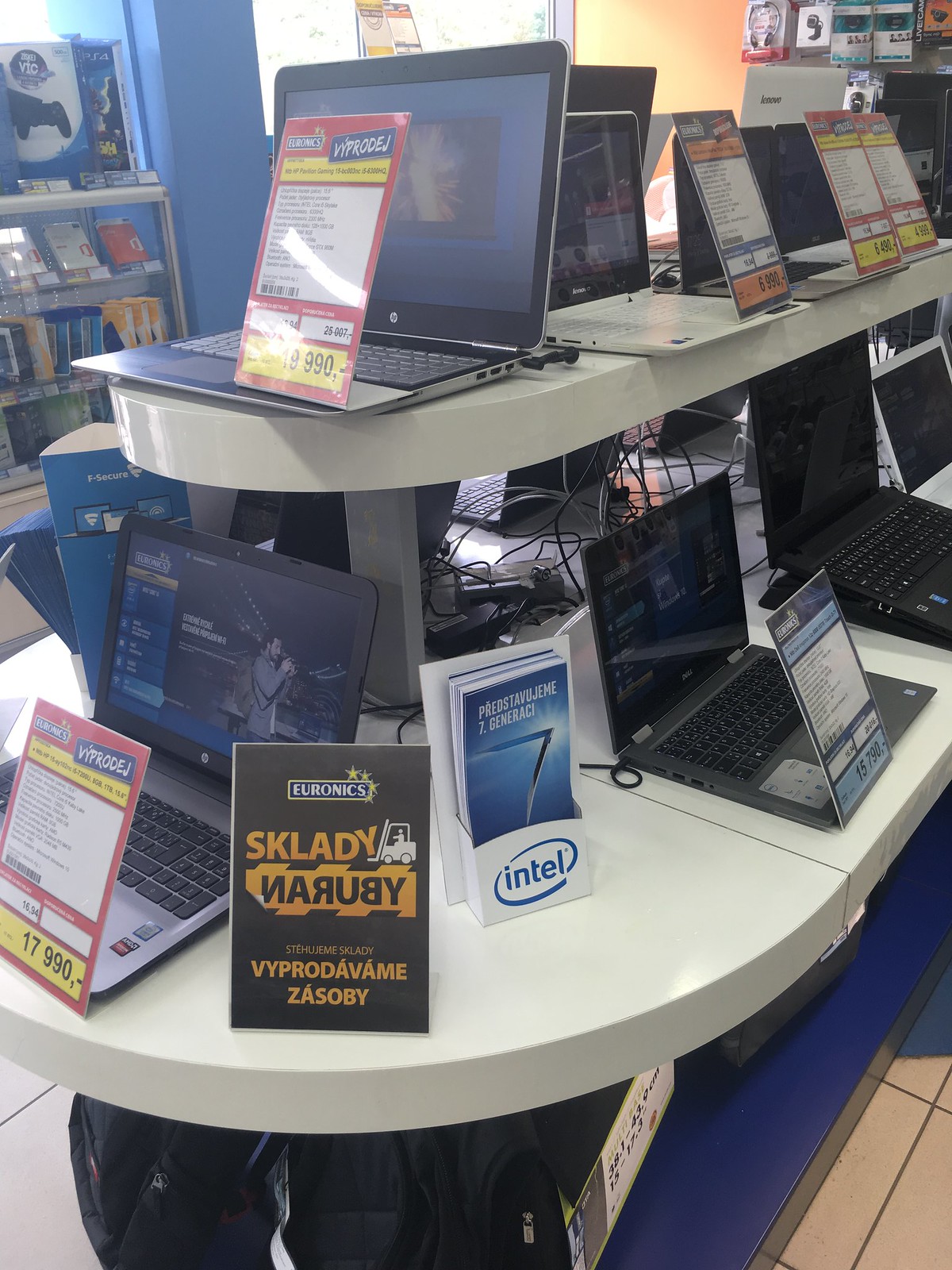This photo captures the interior of an electronics store, possibly called Euronics, given the promotional displays. At the forefront of the image is a two-tiered display counter primarily showcasing various laptops. The main counter, prominently situated towards the lower left, extends out in a rounded peninsula shape and supports a smaller, similarly-shaped tiered counter atop it. This tiered arrangement provides an organized setup where laptops are displayed in two rows, each facing opposite directions, and includes smaller stand-up signs detailing their features and prices – all written in a European language, possibly Polish, Russian, or Hungarian.

At the end of the lower peninsula, a distinctive display features a white compartment holding Intel brochures, marked with the familiar Intel logo in blue. Surrounding the central display are additional counters and shelves. The back left area of the store showcases various electronics and software, including video game systems, while the back right highlights assorted computer accessories, such as webcams and headphones, all hanging in plastic clamshell packaging.

The store's vibrant interior is painted blue and orange and is well-lit, aided by large glass windows allowing ample natural light to stream in. A blue mat under the counters contrasts with the tiled floor, contributing to the overall bright and clean ambiance of the space. Posters and hanging displays further enhance the store's advertising efforts, offering customers a clear view of the diverse electronics available for purchase.